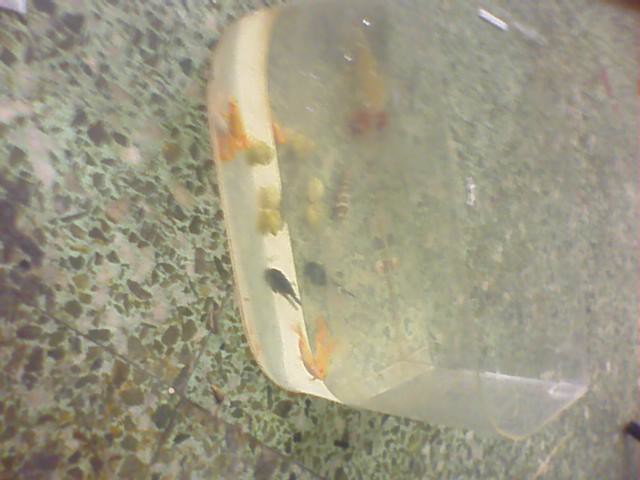The image depicts a somewhat blurry, diagonal close-up of a small fishbowl placed on a muted, floral-patterned tile surface. The tiles are primarily gray, beige, and olive green in color, with elaborate designs resembling leaves in shades of dark green and reddish-brown. Inside the clear, square fishbowl, there is a variety of fish: distinctly visible are two goldfish, one black fish, two green fish, another goldfish, a striped brown and white fish, a yellow fish, and a red fish. The background appears slightly out of focus, further contributing to the blurry and tilted nature of the photograph.